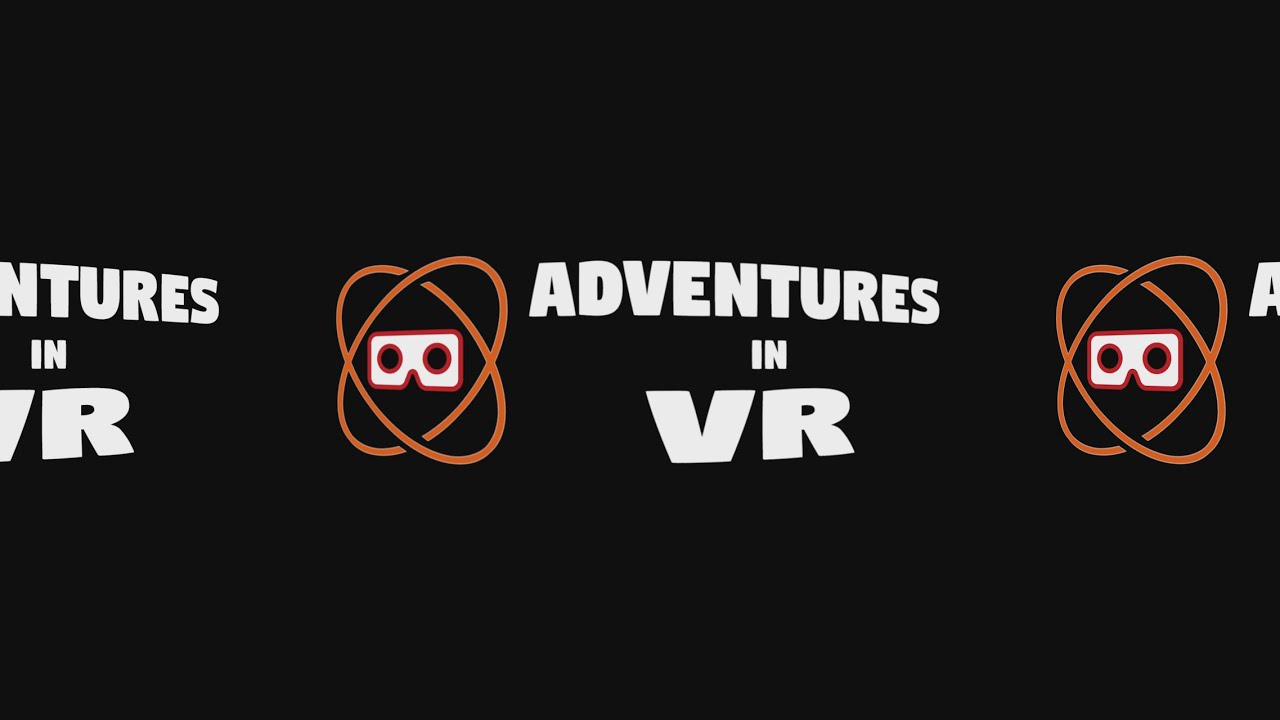The image features a sleek poster with a dark black background, reminiscent of a high definition television aspect ratio. Dominating the center of the poster is the phrase "Adventures in VR" in bold white text. On either side of this text is an orange symbol resembling a nuclear sign with interlocking oval circles, featuring a white mask-like design in the middle, possibly representing a VR headset. This pattern of text and symbol repeats, suggesting a continuous design that extends beyond the borders of the poster. The VR text stands out in bold capital letters, emphasizing the virtual reality theme of the sign. The entire composition is minimalistic yet striking, with the repeating elements creating a sense of depth and continuous adventure in the world of VR.